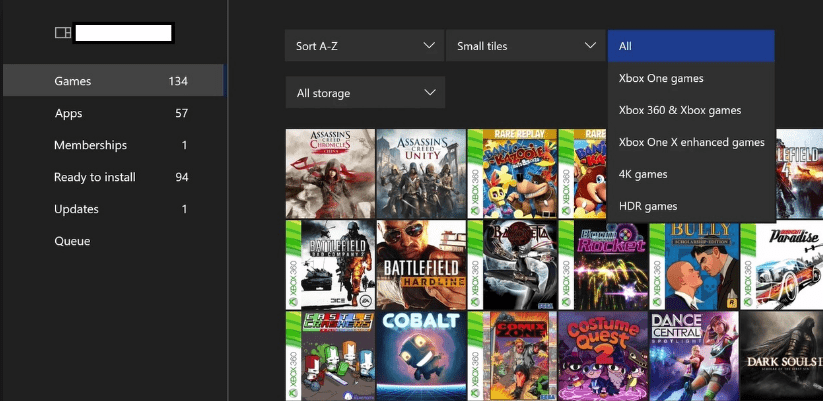The image displays a section from a digital game library interface, featuring a sleek black and gray background. In the top left corner, there's a prominent search bar for locating games, apps, memberships, and related items. Below the search bar are several clickable tabs, each indicating a category and the number of items within it: "Games" (134), "Apps" (57), "Memberships" (1), "Ready to Install" (94), "Updates" (1), and "Queue."

The main section of the interface is segmented to display different organizational features. At the top, there's a drop-down menu labeled "Sort A through Z," adjacent to another drop-down for "Small Tiles." To the right, a third drop-down menu is expanded, showing categories like Xbox One Games, Xbox 360 and Xbox Games, Xbox One Enhanced Games, 4K Games, and HDR Games. Below the sorting options is an "All Storage" drop-down menu.

The games are displayed in a grid format consisting of 6 rows and 3 columns. The first game listed is "Assassin's Creed." Following a top-to-bottom, left-to-right order, the games are: "Assassin's Creed," "Battlefield," "Castle Crashers," "Assassin's Creed Unity," "Battlefield Hardline," "Cobalt," "Rare Replay," an unidentified comic-like item, "Rocket," "Costume Contests," "Bully," "Dance Central," "Battlefield Paradise," and "Dark Souls."

This detailed view provides a comprehensive overview of the user's game library and related categories, each easily accessible through the well-organized interface.